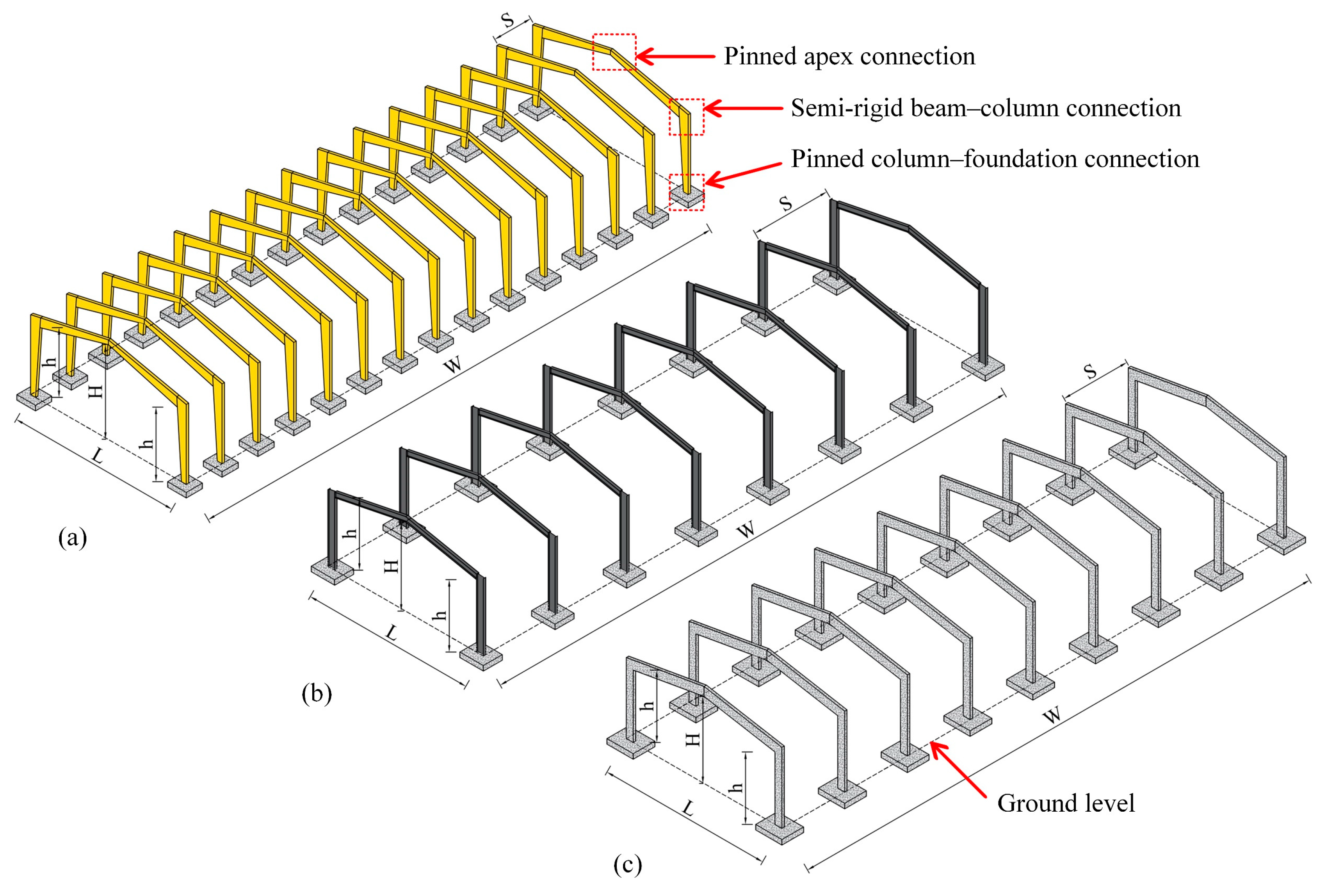This image is a detailed graphic, likely from an instruction manual, illustrating the assembly of a structure that might resemble a barn or a greenhouse. The graphic is divided into three similar but slightly different sections labeled A, B, and C in lowercase black letters within parentheses, located in the lower left-hand corners of each corresponding image.

Each section presents a distinct design: 
- A (Top Image): Features a gold-colored frame depicting the structure with numerous beams extending upwards from rectangular blocks on the ground, converging at a peaked roof. Labels and red arrows highlight key structural connections, such as the "Pinned Apex Connection" at the peak, the "Semi-Rigid Beam Column Connection" where the beams meet the ground, and the "Pinned Column Foundation Connection" at the end of each beam.
- B (Middle Image): Showcases a black-colored design with comparatively fewer beams. This image also carries the same structural connection labels pointing to similar parts.
- C (Bottom Image): Displays a gray-colored design with a slightly greater number of beams than the black design but less intricate than the gold design. The same labels and connections are indicated with red arrows.

In each section, the detailed red arrows and black text descriptors provide clear guidance on how to assemble the structural framework, specifically focusing on pivotal joints and connections critical for structural integrity.